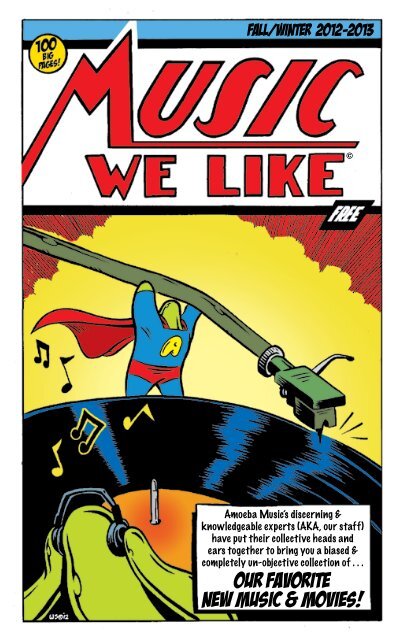This image is a detailed cover of a music magazine titled "Music We Like," styled as a retro homage to the golden age of American comics. At the top left corner, the cover features a yellow circular pop art label with the text "100 BIG PAGES." The top center prominently displays the magazine's title "MUSIC We Like," with the letter 'M' underlining the rest of the word. Below the title, there is a horizontal black bar with small white text boxes, indicating "FALL/WINTER 2012-2013". Dominating the cover is an illustration inspired by the iconic Action Comics No. 1. A muscular figure, reminiscent of Superman but with a green bob for a head and an 'A' on his chest, is holding the arm of a vinyl player. Additionally, on the bottom right, there is text stating "Our favorite new music and movies." In the front, another character is depicted holding headphones. The cover effectively blends nostalgic comic elements with contemporary music themes.